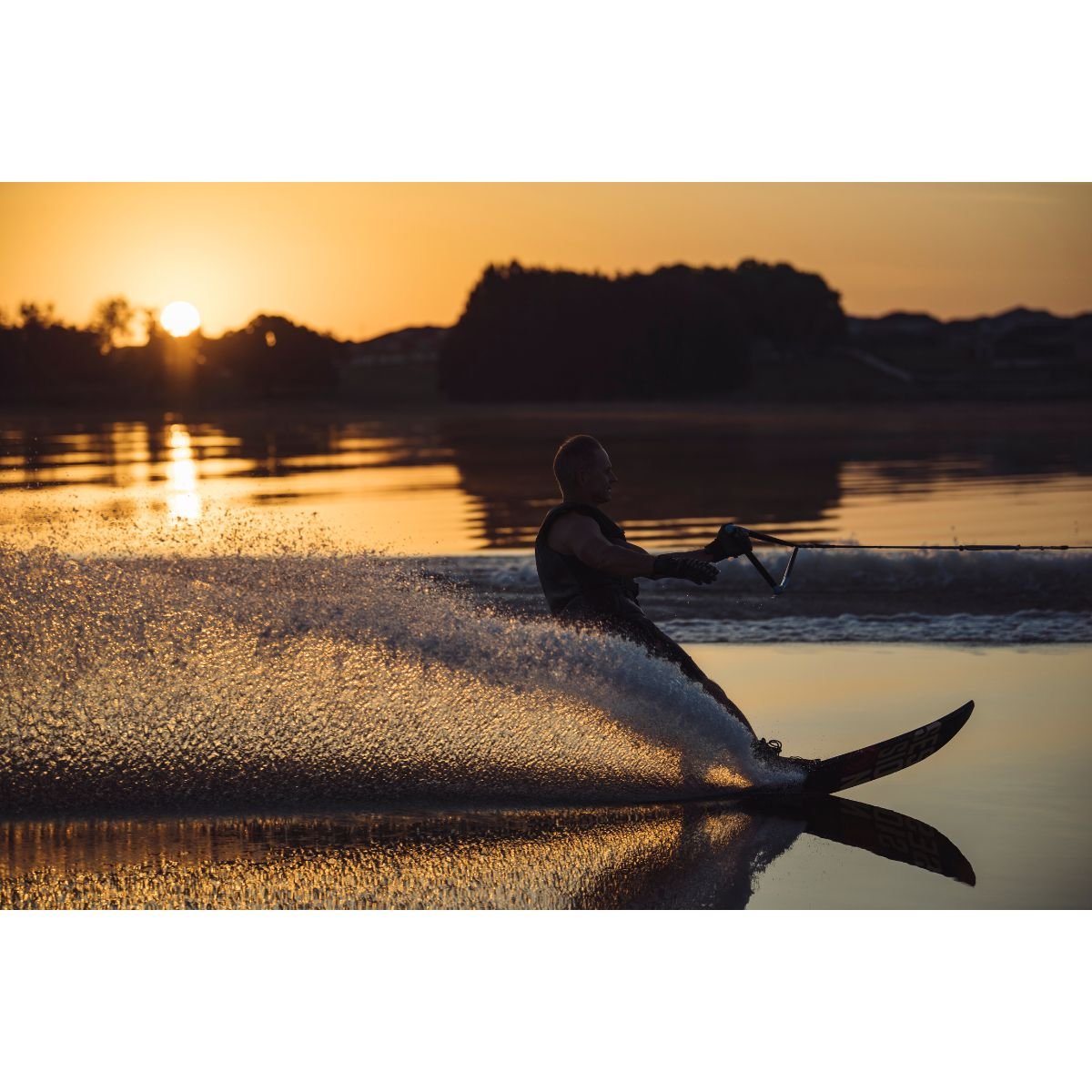The photograph captures a dynamic moment of a man water skiing at sunset. The skier is gliding towards the right on what appears to be a single ski, though the presence of the second ski, if any, is obscured by a jet of water spraying from his ski. This spray partially conceals his lower body. He is leaning back, holding onto a triangular bar with his left hand, his right hand positioned outward for balance. The skier is clad in a wetsuit and a lifejacket for safety. The water ahead of him is remarkably calm, creating a mirror-like reflection of both the ski and the water spray. Behind him, the tranquil water stretches out, reflecting the vibrant orange hues of the sky. The silhouette of trees and hills forms the distant horizon, against which the setting sun peeks just above, casting a warm, golden glow over the scene. The wake of the towing boat trails off to the left, adding a sense of motion to this serene yet exhilarating evening tableau.